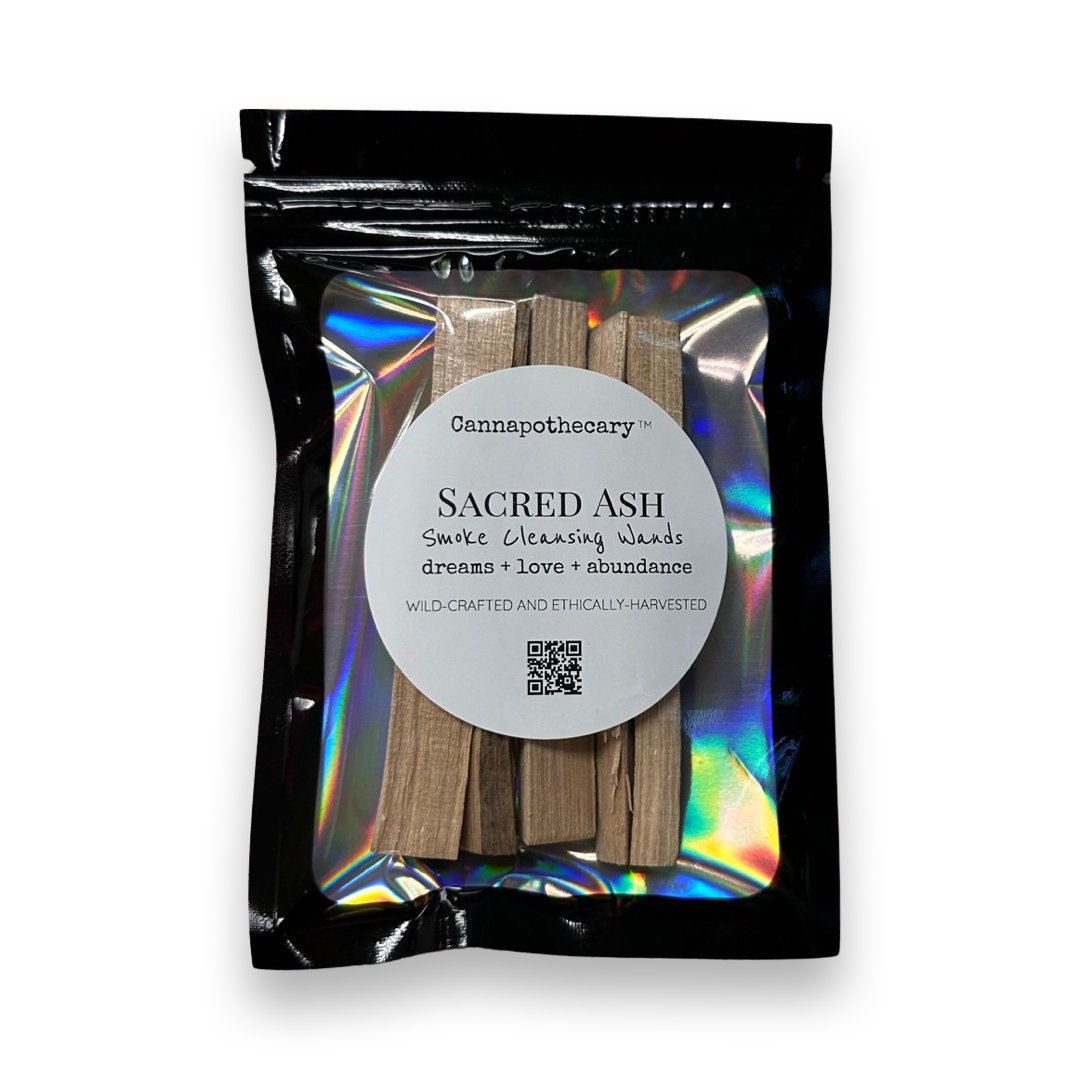The image depicts a black resealable foil bag with a tear-strip, designed for containing incense or smoke cleansing wands. The bag features a clear window on the front, revealing its contents and a mesmerizing prismatic reflective foil on the interior back, which emits rainbow hues. Inside, there are approximately five to six rectangular, flat, greenish-brown sticks, each with a wooden texture and roughly five to six inches in length.

Prominently displayed on the front of the bag is a circular white label with green text. The label reads "Cana Apothecary™," followed by "Sacred Ash" in larger letters. Beneath this, the item is described as "Smoke Cleansing Wands," tailored for "Dreams + Love + Abundance." It is further noted that the wands are "Wildcrafted and Ethically Harvested." The label also includes a QR code at the bottom. The product photo is set against a translucent, transparent background that highlights the bag's shiny, reflective surface.